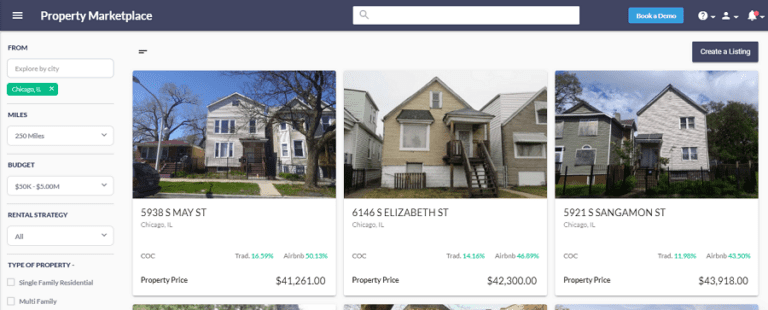Digital Screenshot Description:

The screenshot features a user interface with a purplish header at the top. On the left side of the header, there are three horizontal lines indicating a menu tab, followed by the text options "Property" and "Marketplace." Adjacent to these, there is a white search bar. To the right of the search bar, there is a blue button with white text that reads "Book a Demo." Additionally, there is a white circle containing a question mark, a user profile icon, and a bell icon with a red notification dot.

Below this header, on a white background, the left-hand side displays several interactive filters for a property search. These include:

- A "From" field with a placeholder text "Explore the city" in gray and a green button showing "Chicago IL," indicating Chicago, Illinois.
- A "Miles" filter where the user has selected 250 miles.
- A "Budget" range set from 50K to 5 million dollars.
- A "Rental Strategy" option marked as "All."
- A "Type of Property" category allowing selection of "Single Family, Residency, or Multi-Family," though none appear to be selected.

Further down are images and listings of several properties. The properties include:

1. A white house.
2. A tan house.
3. Another white house.

These properties are priced between $41,261 and $43,918, suggesting the possibility that the screenshot may be from an earlier time, as current market values would likely be higher.